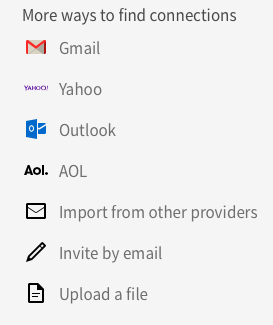The image features a small blue box with the header text "More ways to find connections." Below this header, there are various icons and corresponding text labels representing different email providers and methods to import contacts:

1. **Gmail:** A white envelope with red trim labeled "Gmail."
2. **Yahoo:** A purple icon labeled "Yahoo."
3. **Outlook:** A blue piece of paper and a blue envelope labeled "Outlook."
4. **AOL:** An icon labeled "AOL."
5. **Import from other providers:** A white envelope with a black border labeled "Import from other providers."
6. **Invite by email:** A black pencil with text "Invite by email."
7. **Upload a file:** A piece of paper outlined in black with one corner turned up, labeled "Upload a file."

All of these icons and labels are set against a light blue background, each with its own distinct icon beside the text, visually depicting the various methods available to find and connect with others.